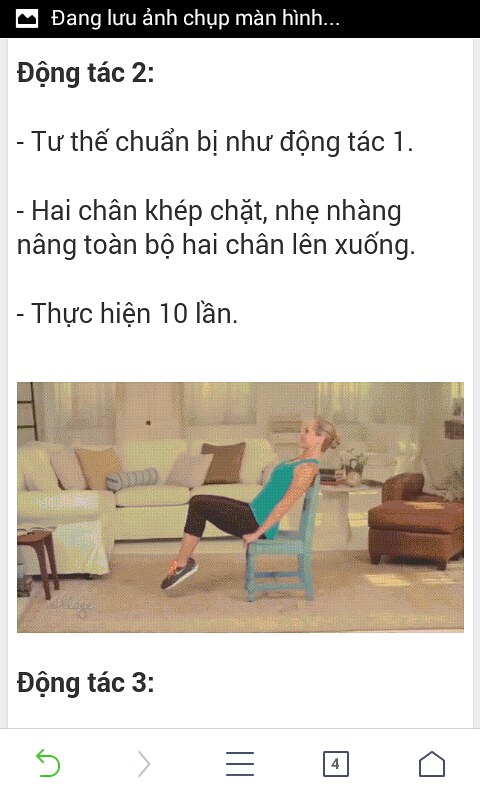This detailed color image appears to show a screenshot of a webpage formatted for a mobile phone, suggested by the visible navigation icons at the bottom, including a green back arrow, a muted grey forward arrow, a hamburger menu, a quadrants icon, and a home symbol, all encased in a thin grey border. The top of the image features a narrow black band with white text in an unfamiliar language, potentially Cambodian or Tagalog. The main content is divided with black text on a white background at both the top and bottom of the screen, also in an unknown language, with the bottom text being slightly bolder.

The central focus of the image is a rectangular photo depicting a blonde woman with her hair in a bun, engaging in what seems to be a yoga exercise. She's wearing a turquoise sleeveless shirt, black leggings, and black-and-white sneakers. The woman is seated on a light blue chair with her feet lifted off the ground, suggesting a yoga or relaxation pose.

The background reveals a cozy living room setting with a pale green sofa adorned with cushions in various colors, including pink, brown, and grey. The carpet beneath her appears to be a mix of green and brown hues. To the left of the scene, there is a yellowish chair or possibly the edge of the couch and a small wooden table. In the upper left corner of the image, part of a ladder is visible, adding to the room's décor. On the right side, there is a brown armchair. The image's overall appearance gives off an impression of a realistically AI-generated art piece.